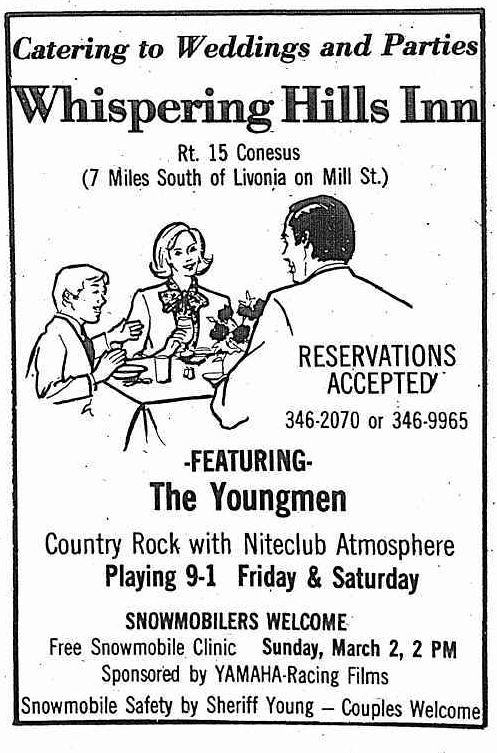This detailed flyer promotes the Whispering Hills Inn's diverse catering services and events. Located at Route 15, 7 miles south of Livonia on Hill Street, the inn offers catering for weddings and parties. The flyer features a black and white illustration depicting a family—comprised of a man, a woman, and their son—seated at a dining table. Highlighted text includes "reservations accepted" with contact numbers 346-2070 and 346-9965.

Additionally, the flyer advertises live music by The Young Men, a country rock band performing with a nightclub atmosphere on Fridays and Saturdays from 9 PM to 1 AM. Whispering Hills Inn also extends a special welcome to snowmobilers and hosts a free Snowmobile Clinic on Sunday, March 2nd at 2 PM, sponsored by Yamaha Racing Films, which includes a snowmobile safety session by Sheriff Young. The flyer emphasizes the inclusion of couples, ensuring all visitors are welcome.